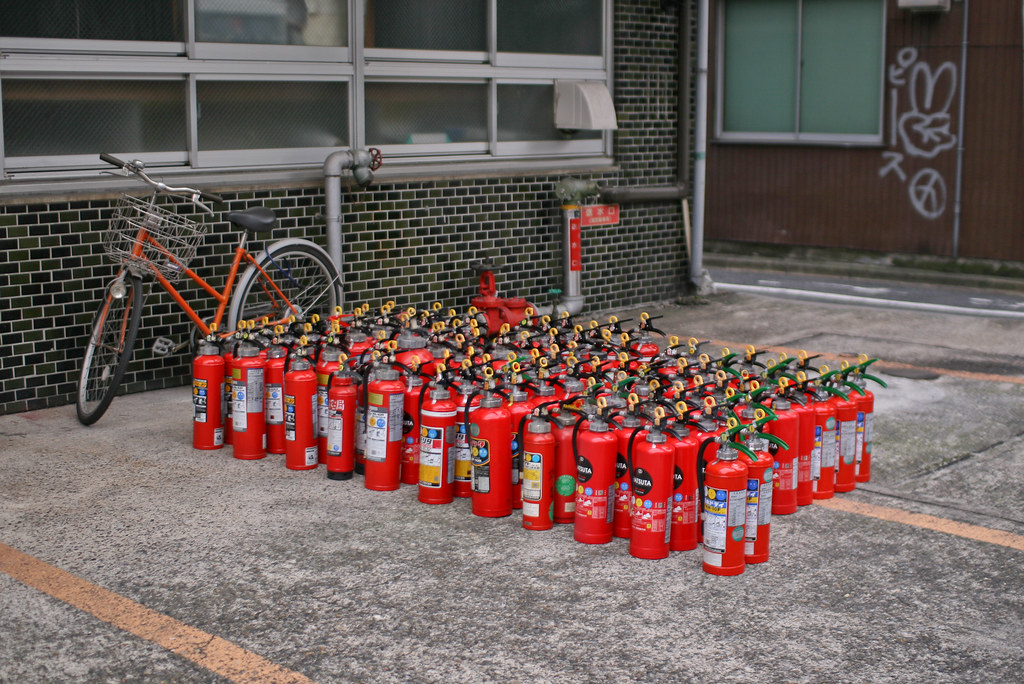In this detailed schoolyard scene, two distinct buildings frame the image. On the top right, there is a burgundy prefab structure marred by graffiti, including a peace sign and various white squiggles. On the left stands a brick building, composed of small, dark, occasionally red bricks that give it a unique appearance. The facade features several pipes and water mains, suggesting part of a fire suppression system. 

In the foreground, an old-fashioned ladies' bicycle with a red frame, white-wall tires, and a front metal basket is parked on its stand. Surrounding this bicycle, on the concrete surface marked with faded yellow parking lines, are rows upon rows of red fire extinguishers. Each extinguisher, slightly different in design, has black and yellow tops and variously colored labels. Organized meticulously, the approximately 120-150 fire extinguishers are arranged in lines, likely ten per row, forming a striking pattern on the ground.

This photograph captures a curious and somewhat chaotic arrangement against the backdrop of an ordinary school setting, drawing attention through its blend of mundane details and unexpected elements.